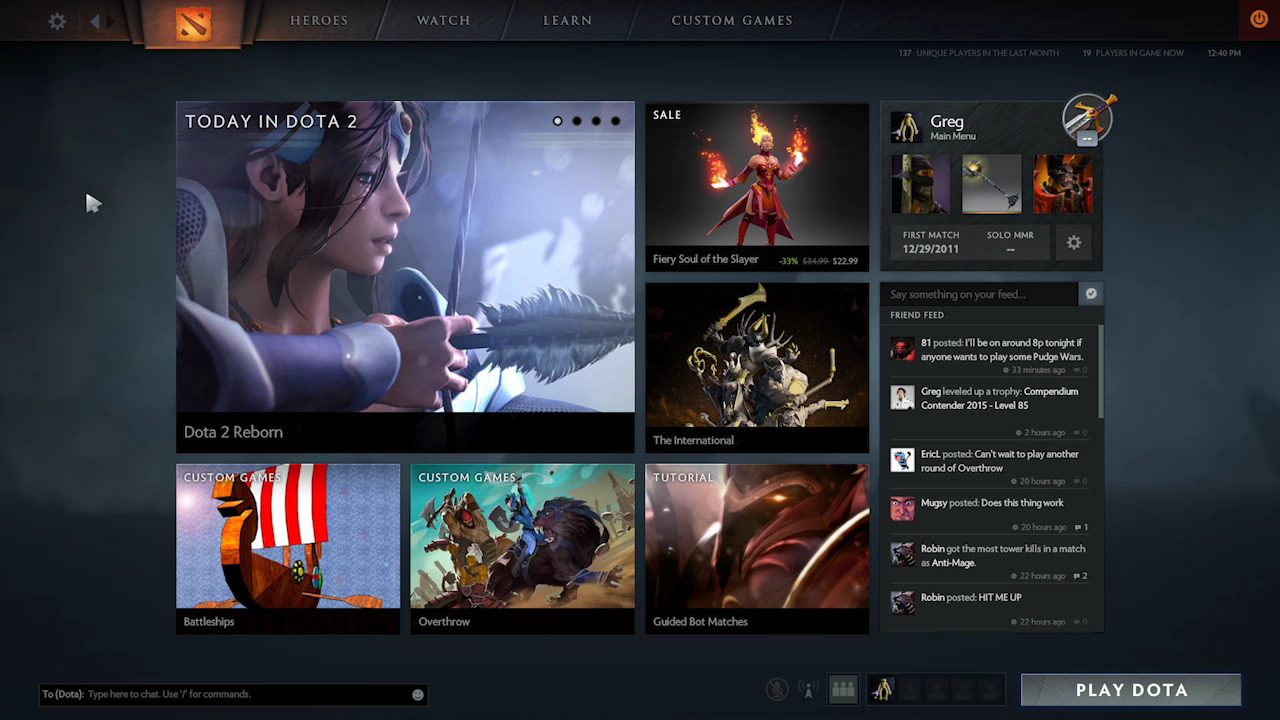The image appears to be a screenshot from the main menu of the game Dota 2. In the bottom right-hand corner, the text "Play Dota" is prominently displayed. At the top, a large tile titled "Today in Dota 2" features an image of a Native American girl with long hair, dressed in a purple outfit, pulling back a bow. The tile also highlights "Dota 2 Reborn". There are three dots in the top corner, indicating a slideshow with the first dot highlighted, suggesting there are likely four more images in the series.

Below this, a promotional banner announces a sale: "Fiery Soul of the Slayer" is available at 33% off for $22.99. The user named Greg is currently viewing his main menu, identifiable by his sword avatar. His profile highlights his first match played on December 29, 2011, and the word "Solo" next to a gear icon, indicating his solo play settings. His profile box also contains several small tiles.

The interface includes a friend feed titled "Say Something on your feed," where updates from his connected friends are visible. Various sections of the main menu are shown, including "The International," "Battleships," "Custom Games," "Overthrow," and a tutorial for "Guided Bot Matches." Multiple pictures are scattered around the interface, enhancing the visual complexity. The upper left-hand corner features a gear icon, and across the menu, there are navigational paths titled "Heroes," "Watch," "Learn," and "Custom Games."